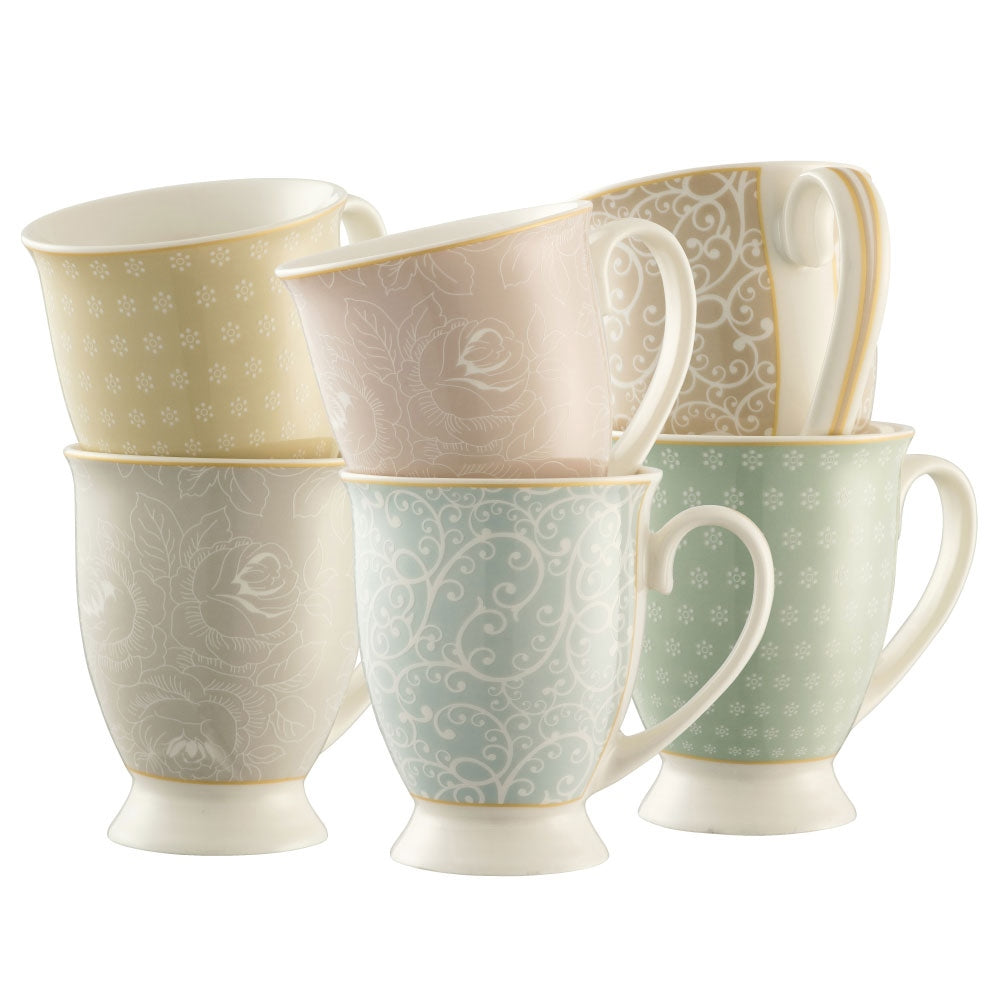This detailed photograph features six elegant teacups arranged in two stacked rows, set against a pristine white background. The cups are presented in pastel colors, each adorned with delicate patterns. The bottom row displays a variety of designs: 

- On the left, a beige-gray teacup with white roses, gold accents at the rim and base, and a white handle.
- In the center, a soft blue teacup featuring intricate white filigree and swirls.
- To the right, a soft green cup decorated with small white starburst flowers.

Stacked inside each of these bottom cups are matching colorful counterparts:

- Inside the beige-gray cup is a buttery yellow teacup with small white flowers.
- Nestled within the blue cup is a pale pink teacup with white roses.
- Inside the green cup is a tan teacup adorned with a white swirly pattern and a handle with gold stripes.

These teacups, with their consistent white handles and bases, and their delicate, ornate designs, capture a sense of refined elegance and harmonious color coordination.